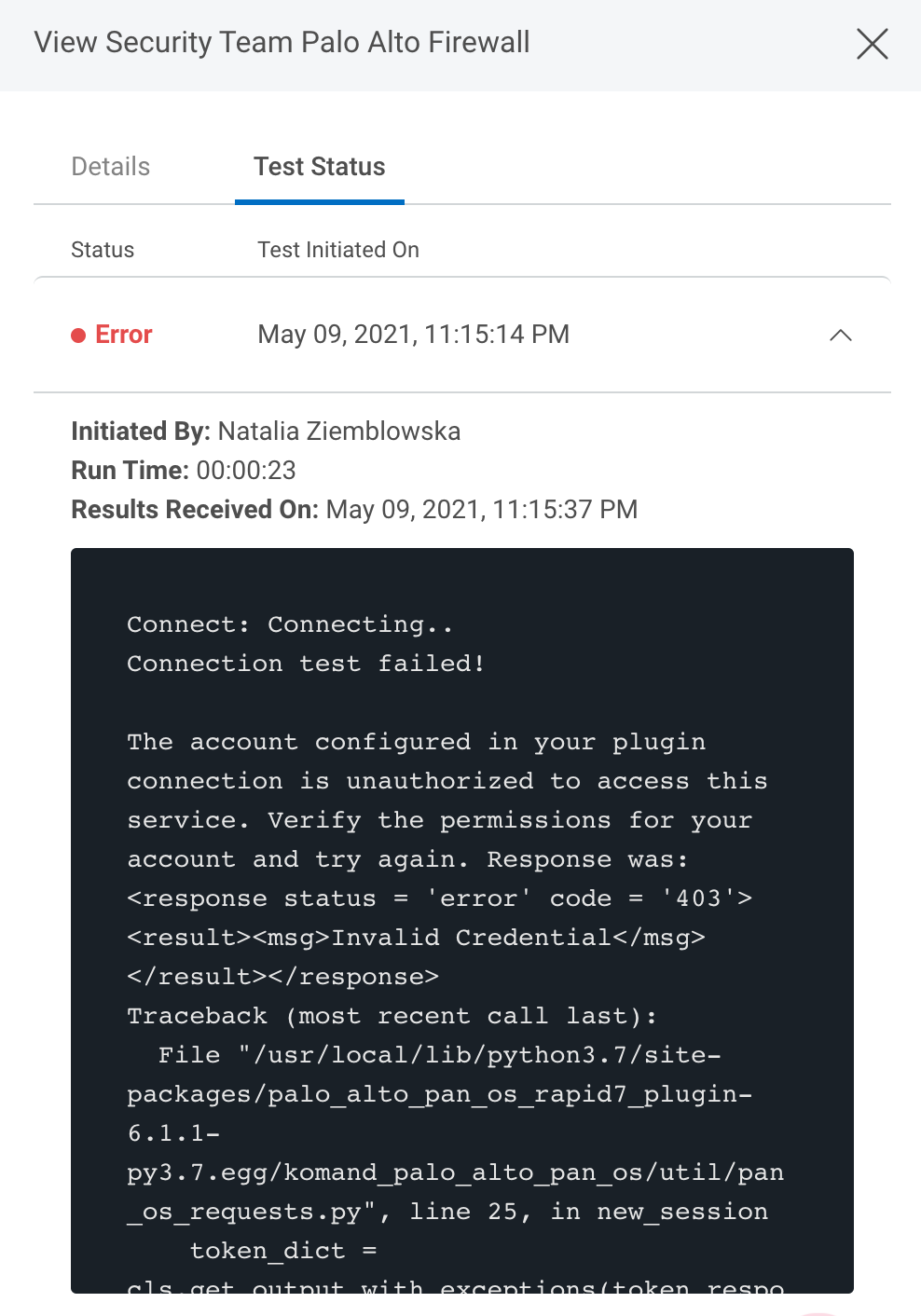A screenshot with a white background showcases a gray rectangular interface detailing a recent security test. The interface includes several key elements:

- **Title**: "New Security Team Payload"
- **Labels**: "Auto," "Firewall" (marked with an "X"), "Details," and "Test Status" all presented in black text.
- **Status**: Marked with a red circle indicating an error.
- **Test Initiation**:
  - Timestamp: May 9th, 2021, 11:15:14 p.m.
  - Initiated by: Natalia Zemblowska
  - Runtime: 00:00:23
- **Results Reception**:
  - Timestamp: May 9th, 2021, 11:15:37 p.m.
  
A message indicates a connection test failure:
- **Error Message**: 
  - "The account configured in your plug-in connection is unauthorized to assess this service. Verify the permissions for your account and try again."
  - Further details include a response code stating: 
    - "Response status = 'error' code = '403'"
    - An additional message indicates: 
      - "Result: Invalid Credential"